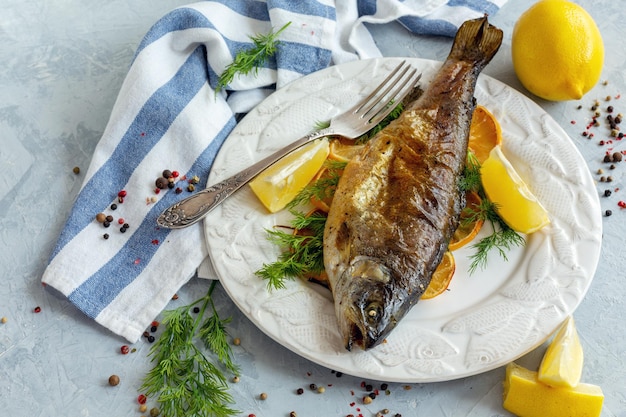The photograph captures a clean, crisp indoor setting with a focus on a round, white embossed plate featuring a whole poached fish, possibly a trout, displayed prominently at its center. The fish, charred with a crisp brown skin, lies with its head facing downward and its tail extending off the plate. Around the fish are lemon wedges and a bed of oranges and dill. A silver fork rests on the left side of the plate. The plate itself is detailed with embossed fish shapes on its gray-edged rim. The backdrop includes a white and blue striped towel to the left, with mixed peppercorns—red, white, and black—scattered across a light gray marble-like tabletop. Additional elements include a whole lemon positioned at the top right of the plate and some more dill sprinkled around, contributing to the bright and immaculate presentation of the scene.